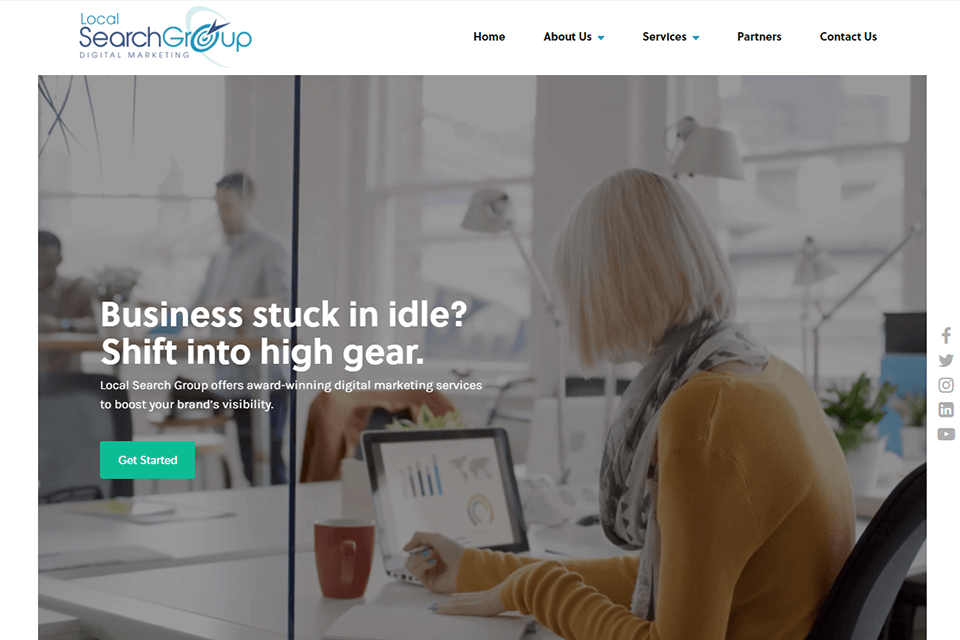Screenshot of a web page for Local Search Group’s digital marketing services, prominently featuring their tagline “Business Stuck and Idle? Shift into High Gear.” The page header includes navigation tabs for Home, About Us, Services, Partners, and Contact Us.

The page is dominated by a large, slightly blurred indoor office scene, with a gray overlay. In the foreground, a woman wearing a yellow top and a large scarf is seated at a white desk, focusing on her computer screen. Her left side and back are partially visible as she keeps both hands on the desk, with a coffee mug nearby. The modern office space is well-lit by contemporary white desk lamps.

In the background, a man stands next to another seated man, engaged in conversation. A chair with a jacket draped over it and a desk with a potted plant add to the bustling office environment. The windows on the far right side reveal a view of neighboring office buildings. Overlaid on the image is text promoting Local Search Group’s award-winning digital marketing services with a call-to-action button labeled "Get Started."